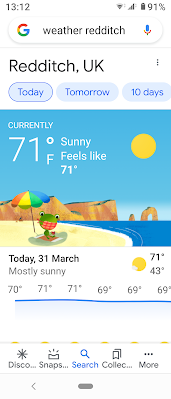This screenshot depicts a mobile weather application interface. At the top, the status bar shows the current time as 13:12, alongside a Wi-Fi symbol, a battery icon indicating 91% battery life. Below it, a Google search box is displayed with its signature colors: red, gold, green, and blue. In black text, it reads "Weather, Redditch" and includes a microphone icon in blue, gold, and red, denoting voice search capability. The location is specified as Redditch, UK, with three gray dots arranged horizontally beneath it.

Following this, there are three blue buttons: "Today," "Tomorrow," and "10 days." Below these buttons, in white font, it states the current weather conditions: 71 degrees Fahrenheit, sunny, and feels like 71 degrees. Next to this text, there's a gold sun icon.

The screen features a whimsical cartoon image of a green frog with big, white googly eyes, wearing a red and white plaid mask, relaxing on a white sandy beach under an orange, gold, green, and blue beach umbrella. The frog sits on a red and white towel, with blue water visible in the background.

Further down, the screen displays the date, "Today, 31st March," next to a sun icon, with the weather described as "mostly sunny." Temperature predictions are listed as 70, 71, 71, 69, 69, 69 degrees Fahrenheit, with a high of 71 and a low of 43.

At the bottom of the image is a white bar featuring a series of black icons labeled: "Discover" with a sparkle icon, "Snapshot" with a box icon, "Search" with a blue magnifying glass, "Collections" with a ribbon icon, and "More" with three gray dots. There is also a gray back arrow and a gray bar. This sums up the key elements of the screenshot.